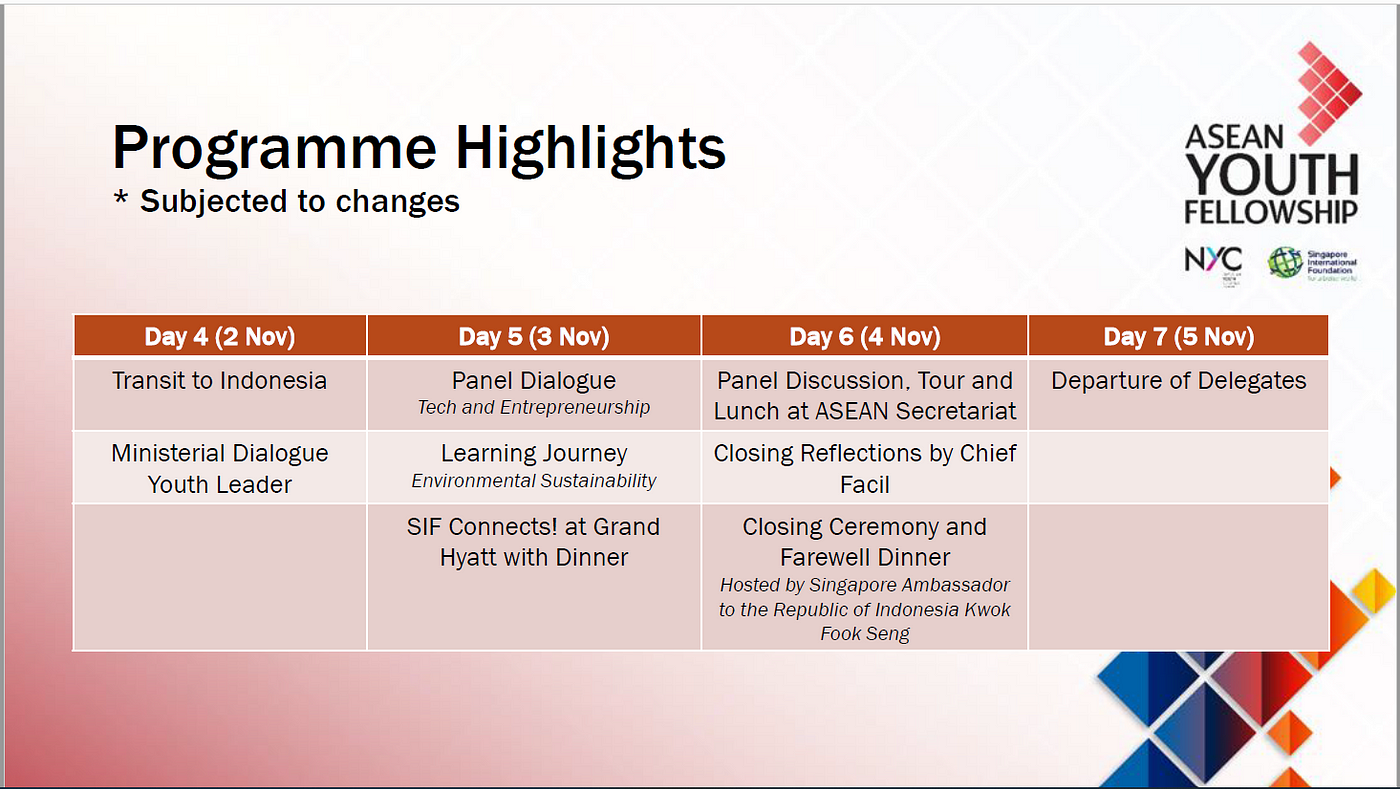The advertisement showcases a detailed schedule for the Eshaan Youth Fellowship, NYC program. The top half of the background is white, featuring "Program Highlights" in black text, followed by "Subjected to Changes." In the top right corner, a red arrow made of small boxes points to the right. Below, the program, displayed in a grid format, details events from Day 4 to Day 7 with columns labeled accordingly: Day 4, 2 November; Day 5, 3 November; Day 6, 4 November; and Day 7, 5 November. 

For Day 4, the events include "Transit to Indonesia" and "Ministerial Dialogue Youth Leader." Day 5 outlines a "Panel Dialogue," "Learning Journey," and "SIF Connects at Grand Hyatt" with dinner. Day 6 features activities like a panel discussion, a tour and lunch at ASAN Secretariat, closing reflections by Chief Faisal, and a closing ceremony and farewell dinner hosted by Singapore’s Ambassador to Indonesia, Mr. Kwok Foon Seck. Finally, Day 7 marks the "Departure of Delegates." This multi-day event promises an engaging and immersive experience for participating youth leaders.